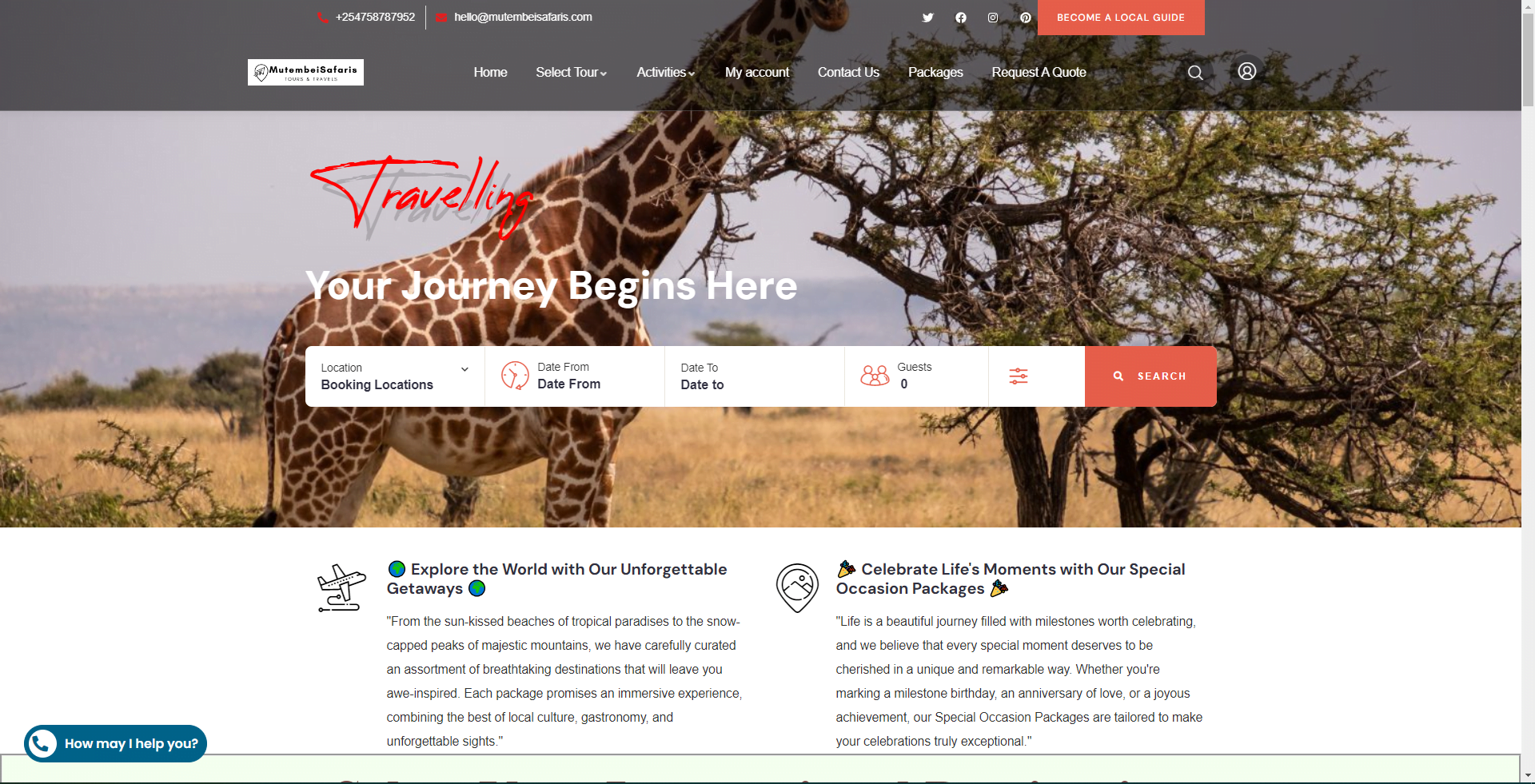In this horizontally rectangular image, which appears to be a screen grab from a touring website, the upper portion and upper two-thirds of the background showcases a giraffe engaging in the natural behavior of chewing on a short tree. This scene is set against a backdrop of a landscape filled with high, dry grass.

Overlaying this serene wildlife image, in the top right corner, there is a prominent orange button labeled "Become a Local Guide." Below this button, centered horizontally across the image, is a navigational menu with various page options: "Home," "Select Tour," "Activities," "My Account," "Contact Us," "Packages," and "Request a Quote."

Underneath the menu, a motivational phrase "Traveling: Your Journey Begins Here" is prominently displayed, indicating the adventurous spirit of the website. Just below this phrase, there is a narrow horizontal banner labeled "Booking Locations," which includes a drop-down menu for selecting travel details such as "Date From," "Date To," and "Number of Guests." Accompanying these fields are a filter icon and a search icon, providing users with tools to refine their travel plans.